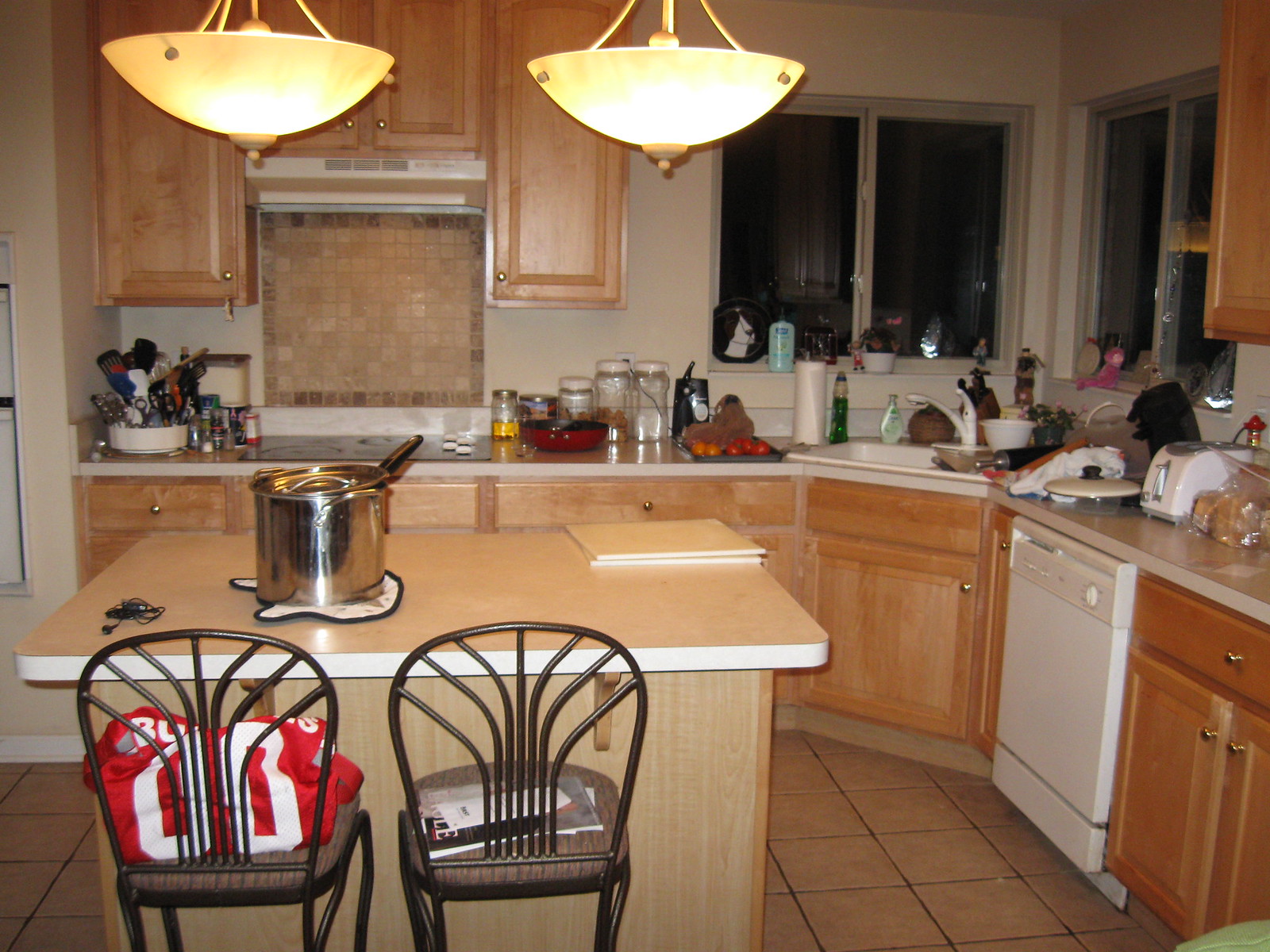This image depicts a homey kitchen with a cozy and functional layout. The back walls are adorned with brown cabinets, providing ample storage space, and there are two cabinets mounted above a stove on the left side of the image. Positioned on the countertop directly below the cabinets is a large, indistinct square object. To the left on the counter, there's a pot filled with utensils.

Moving to the right, several jars of flour or flavorings are neatly arranged, with some fruit visible nearby. This section of the wall features two windows, and where the wall bends, there are two additional windows bathing the sink with natural light, which is nestled in the corner. Above and below the countertop, more brown cabinets line the space, ensuring plenty of storage for kitchen essentials. The countertop itself has a light brownish-gray hue.

Adjacent to the sink is a white dishwasher. Positioned above the dishwasher, a toaster is surrounded by various miscellaneous items. 

In the center of the room stands an island that matches the color scheme of the countertops and cabinets. A pot with utensils sits on a pot holder in the middle of the island. Two chairs flank the island: the left chair holds a red piece of clothing, while the right chair has a booklet or magazine resting on it. This kitchen scene combines functionality with a lived-in, welcoming feel.